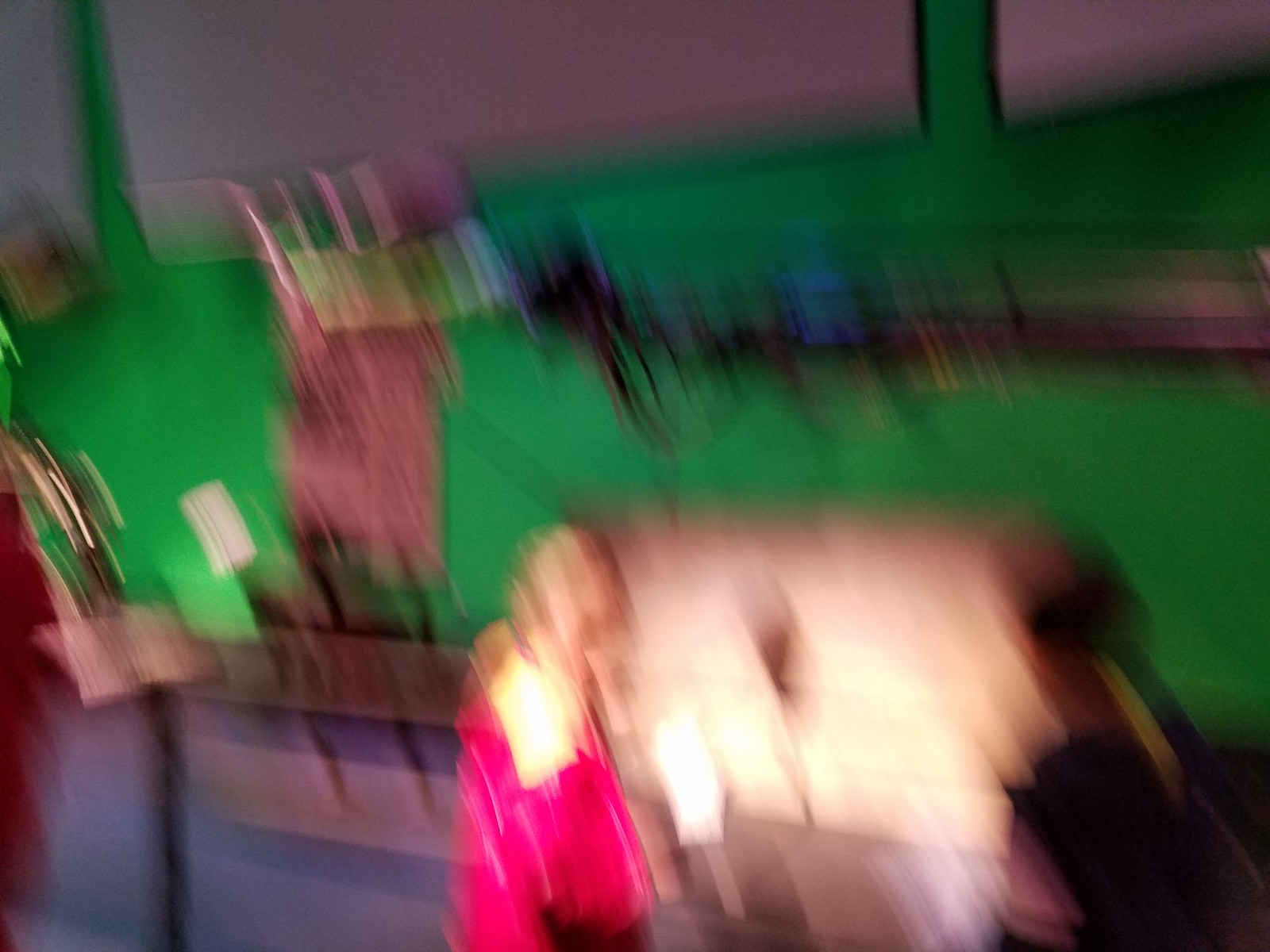In this highly blurry photograph, a woman with blonde hair is discernible in the foreground, either wearing or carrying a bright magenta-colored item of clothing while walking and looking down. To her left, across a brown wooden fence, there is a pale pink object. Beyond the fence lies a large expanse of vibrant kelly green terrain, which contrasts with a section where a bright blue object can be seen in the distance.